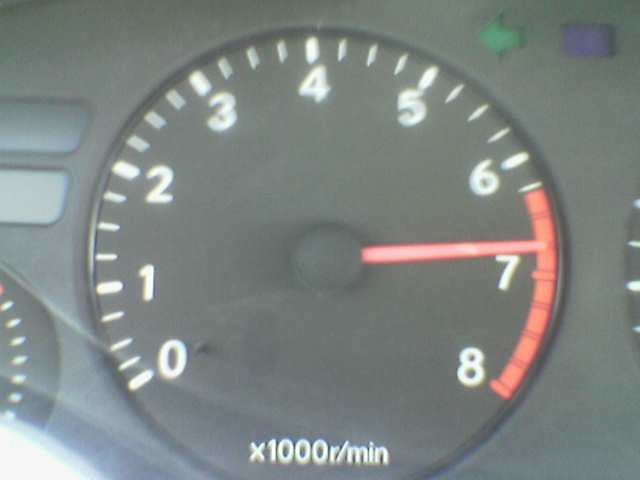A close-up photograph captures a highly out-of-focus tachometer, likely from a car given its range from 0 to 8 RPM x1000. The redline area spans from approximately 6200 RPM to 8000 RPM. The tachometer features a black face with white numerals and a red needle which indicates a current engine speed of about 6600 RPM. This high reading could explain the blur and vibration obvious in the image. In the center of the tachometer is a black circle, while to the left, a partial view of another dial with white markers around its edge is visible. Additionally, at the top right corner of the frame, there is a small green left-turn indicator and a blue rectangular element. On the far right, another dial with four white circumferential marks is partially visible.